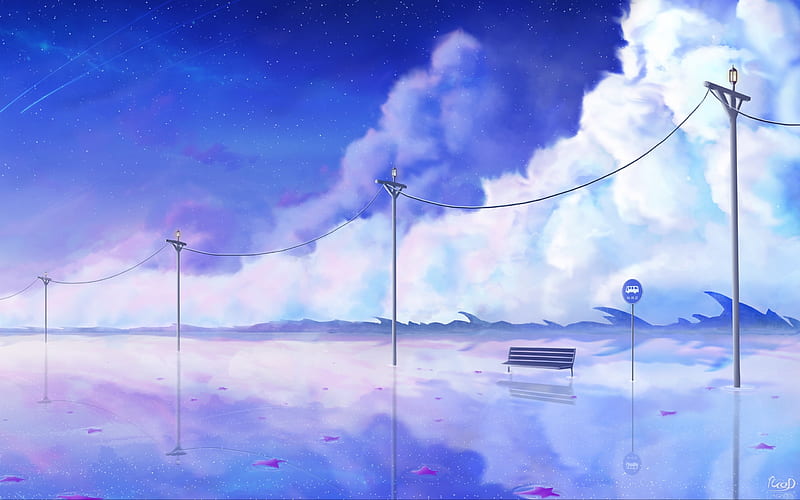This surreal painting depicts a flooded bus stop scene under a complex, vividly colored sky. Central to the image is a bench to the right, with a blue bus stop sign displaying a white bus icon nearby. Above, telephone poles with power lines stretch across the composition, one featuring a light post. The sky transitions from a whitish blue at the clouds in the top right, interspersed with hints of purplish and bluish hues, to a darker dusk-colored blue towards the top with tiny white stars twinkling. Two shooting stars with trailing tails adorn the sky in the top left corner. The setting includes reflective, water-covered ground akin to a flooded road, peppered with whimsical details like purple starfish. Ocean waves crash against a retaining wall in the background, blending with the ethereal ambiance of the piece.